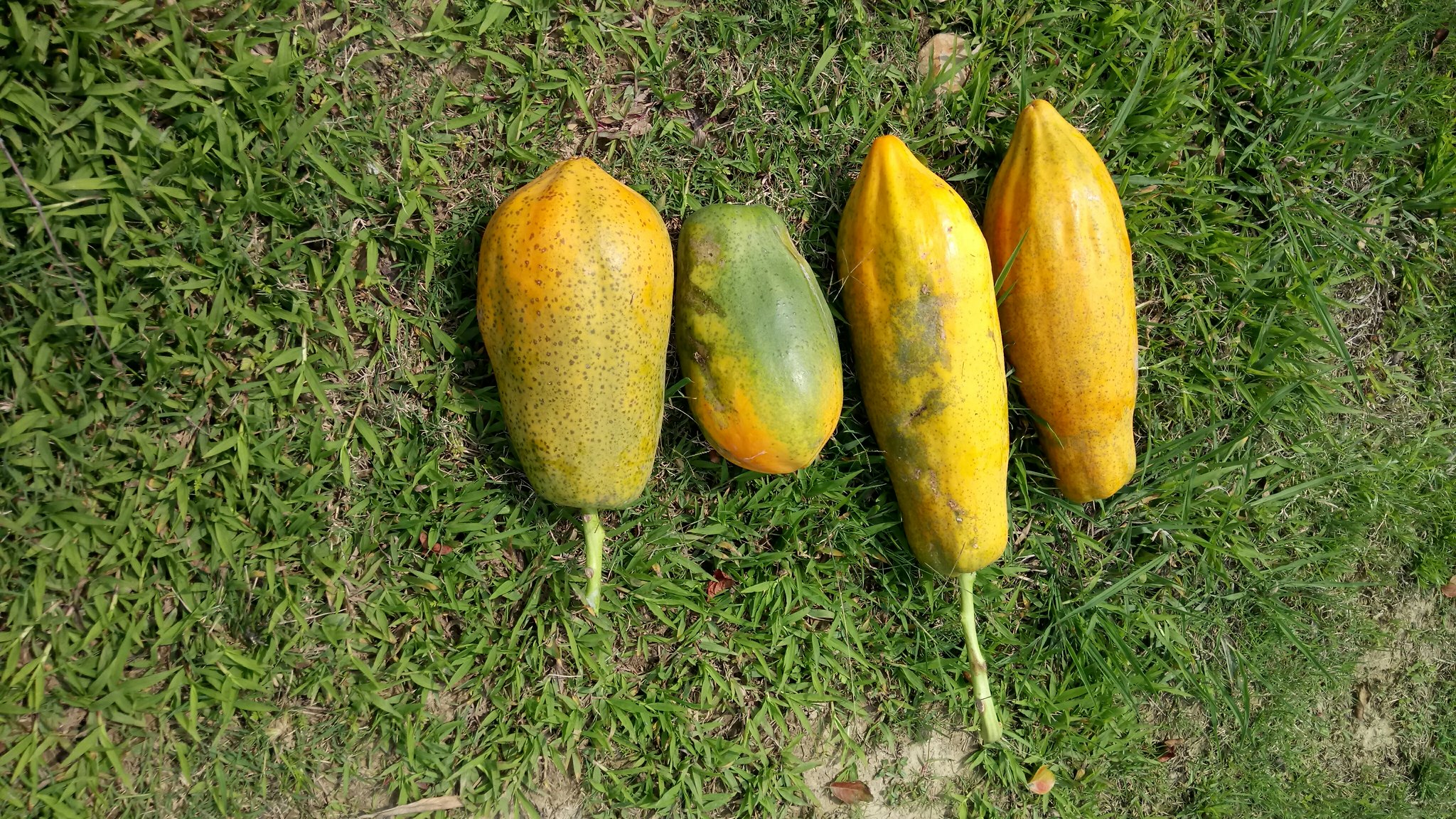The image shows an overhead view of a rough, dry patch of grass interspersed with visible soil patches and dotted with a few brown leaves. On this uneven greenery lie four distinctive, homegrown squash. The squashes display a variety of shapes and colors: the one furthest to the right is elongated like a torpedo and bright yellow; next to it is a similarly shaped squash with a mix of yellow and green hues; the third squash is smaller, somewhat resembling an avocado, and exhibits a green base with patches of rosy tint and yellow; the final squash on the far left has a pear-like shape. All the squashes exhibit a homemade quality, featuring vibrant lemony yellow tones accented with dark green streaks and patches, suggesting they've been freshly picked from an allotment. Some have visible green stems still attached, adding to their fresh, organic appearance.